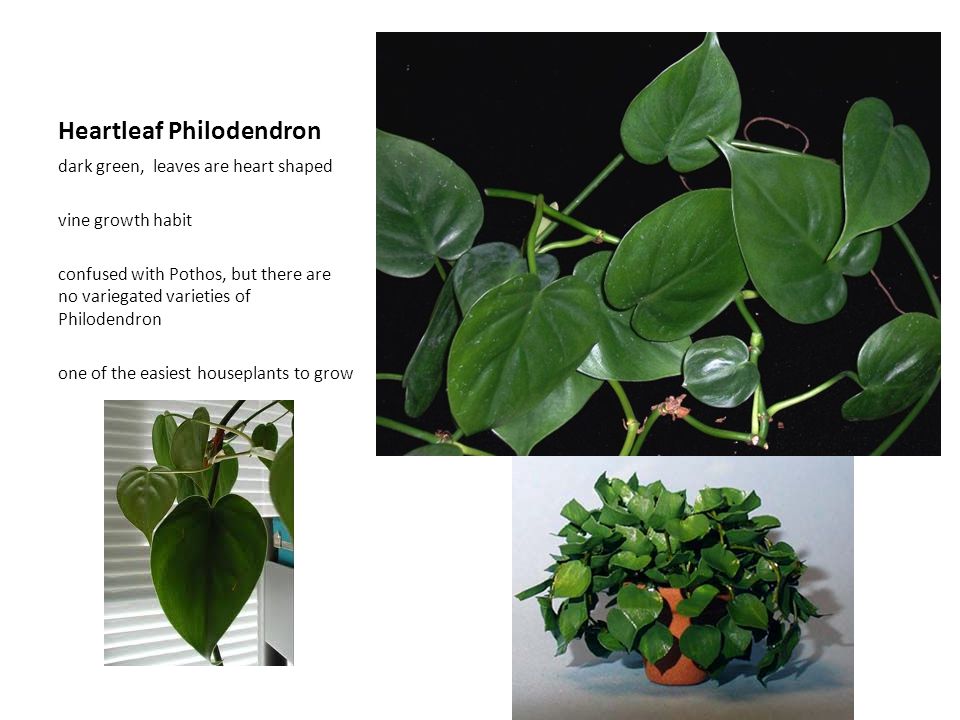This full-color image is a collage featuring three photographs and descriptive text about the heartleaf philodendron, known for its dark green, heart-shaped leaves and vine growth habit. The largest photograph, positioned at the top right, showcases several vibrant leaves set against a stark black background, illuminated by a fluorescent light. Below it, the smallest photograph on the left captures the plant’s leaves draping from white window blinds, adding a touch of greenery to the scene. The centerpiece of the collage features a full view of the philodendron in a terracotta ceramic pot, showing the plant’s lush foliage thriving in an indoor setting. The accompanying text explains that the heartleaf philodendron is often confused with pothos but lacks variegated varieties. Notably, it’s highlighted as one of the easiest houseplants to grow, making it a popular choice for indoor gardening enthusiasts.